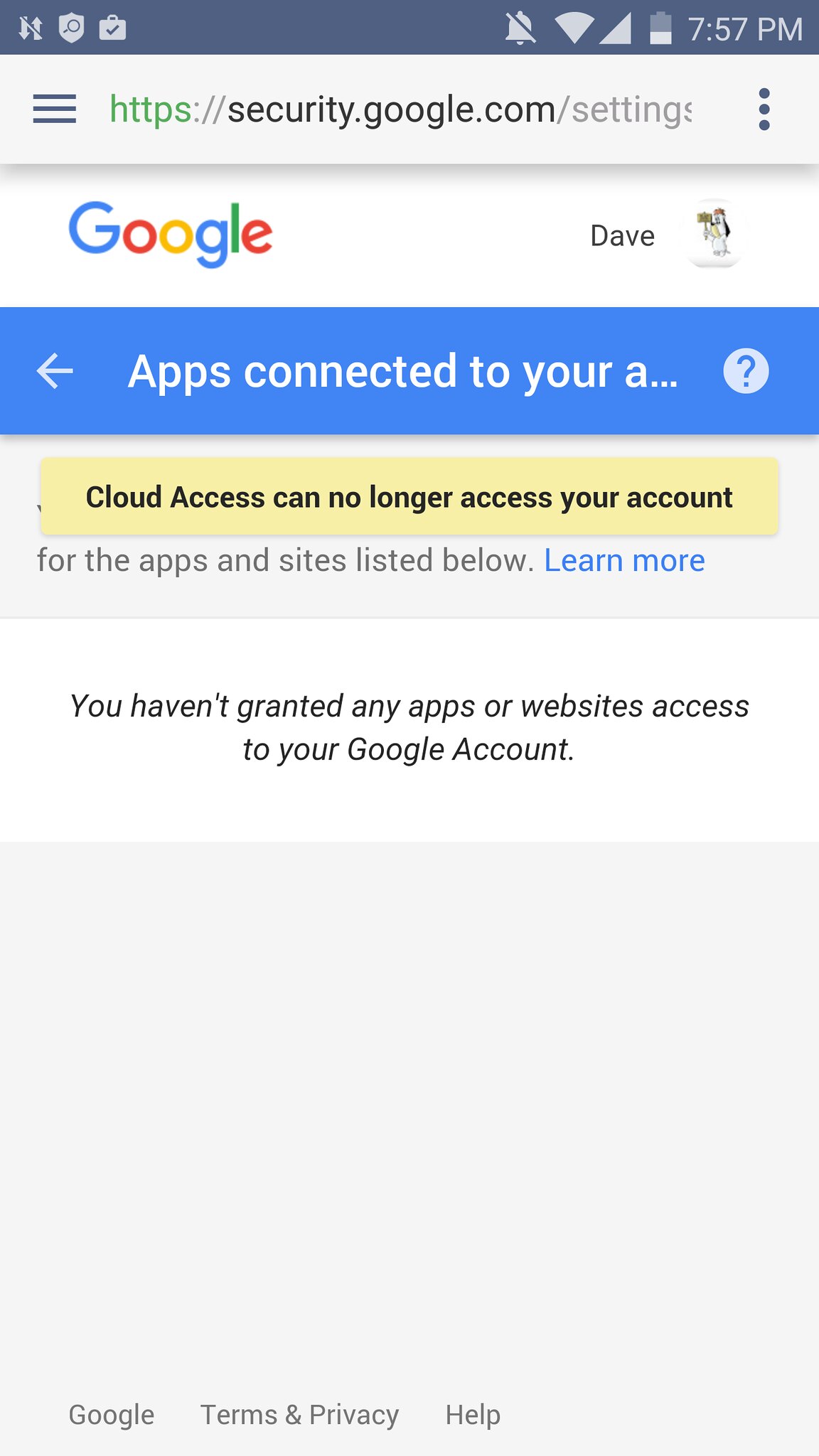This is a detailed screenshot from a mobile phone depicting a Google account security settings page. 

At the top, there is a navy blue status bar showing three notifications in the upper left corner: one with a two-arrow icon, another with a shield and magnifying glass icon, and the third with a briefcase and checkmark icon. 

On the right side of the status bar, there are several icons: a bell with a stripe through it, an upside-down triangle, a sideways triangle, and a battery icon that is two-thirds filled. The time displayed is 7:57 p.m.

Below the status bar, the address bar shows the URL: "https://security.google.com/settings." Next to the URL, there are three horizontal dots indicating additional settings. 

The main content features the Google logo in its characteristic rainbow colors, followed by the name "Dave" in black font and an adjacent icon.

A prominent blue bar below this header reads: "Apps connected to your account have been removed. Cloud access can no longer access your account. You haven't granted any apps or websites access to your Google account." This is a clear indication that no third-party apps or websites have been permitted to access the user's Google account.